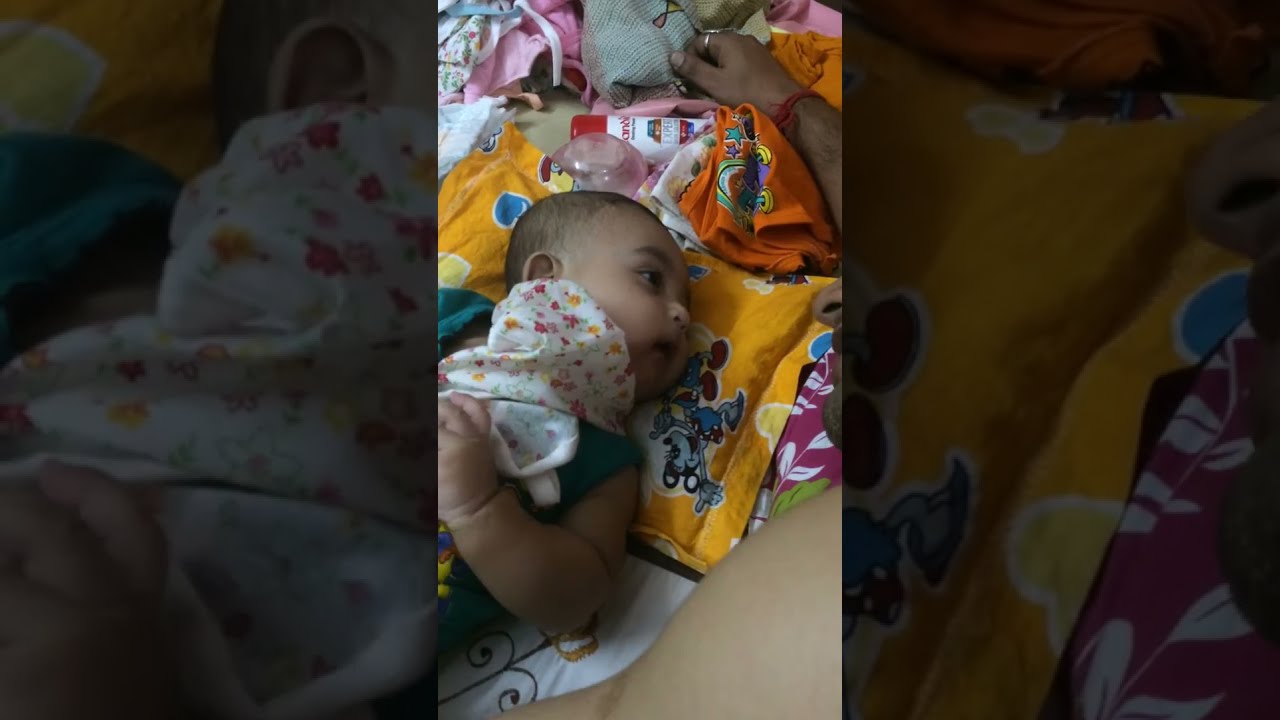This photograph showcases a baby, possibly of African American or Mexican descent, lying on its side with its head resting on a vibrant, golden-orange pillow adorned with blue and yellow hearts and other indiscernible shapes. The baby is dressed in a forest green vest or onesie that features colorful letters spelling "baby sports" and cartoon characters, including one with blonde hair. The baby is holding something white with floral designs in its hands. Surrounding the baby are various pieces of clothing, including folded onesies in shades of orange, white, and pink, which could also be small towels. A pink ball is visible in the background, along with a floral blanket in pink, green, and white hues resting nearby. Vertical black strips appear on either side of the image.